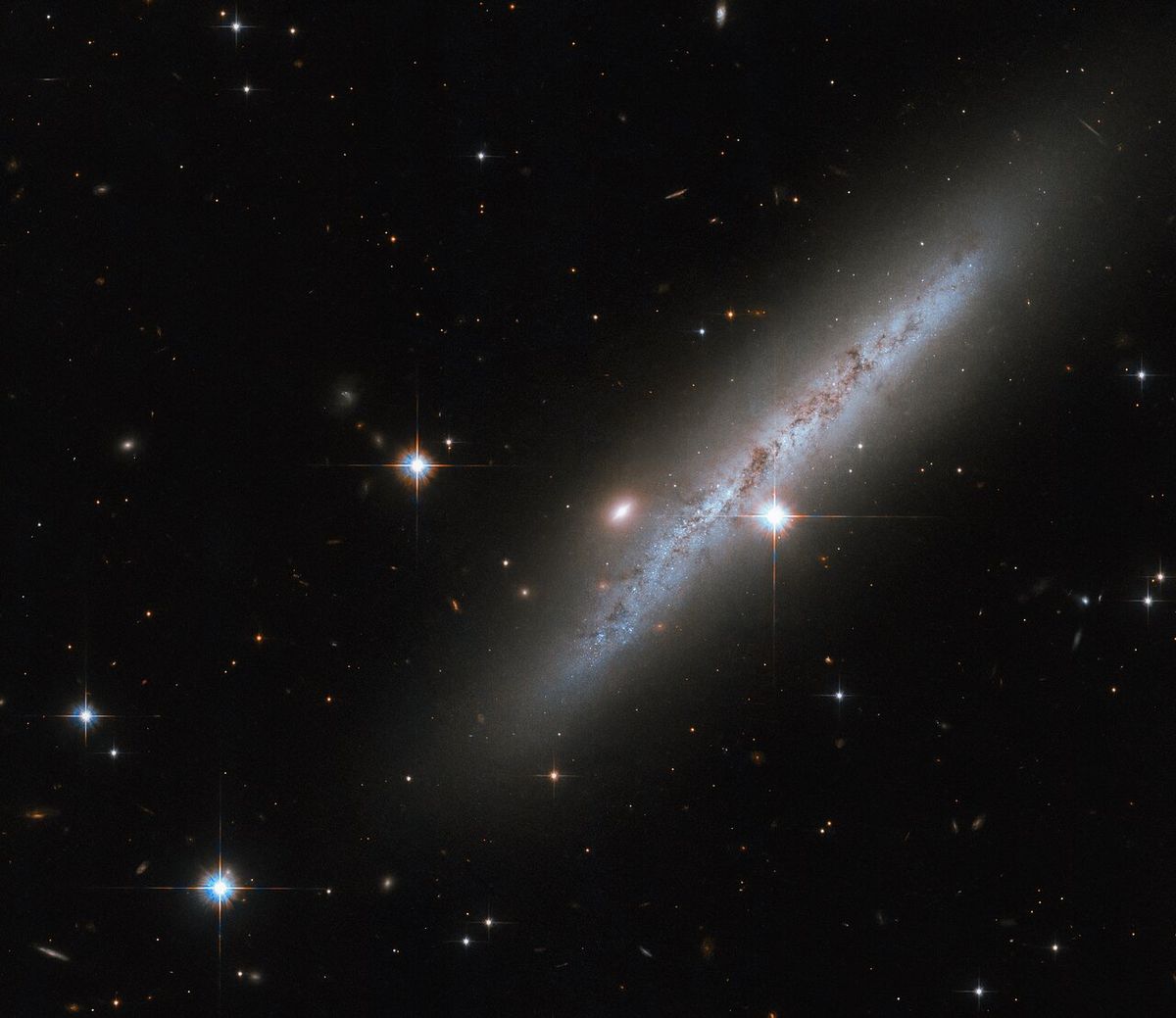This image captures the mesmerizing expanse of the night sky, dominated by a profoundly dark background dotted with countless, scattered stars. Positioned diagonally to the right, a brilliant galaxy stands out as the brightest feature. This galaxy, an elongated oval disk, boasts a rich tapestry of colors, including light blue, reddish-brown hues, and a surrounding aura of whitish, cloudy mist that fades at the borders. The intricate nebula-like structure of the galaxy gives it a mystical and ethereal ambiance. Surrounding this central marvel, various stars of differing sizes pepper the sky. Among them, about five larger stars shine more brightly than the others, contributing to the profound sense of cosmic depth and beauty portrayed in the image. Above and to the left, two notably bright stars can also be seen, adding to the intricate nightscape.